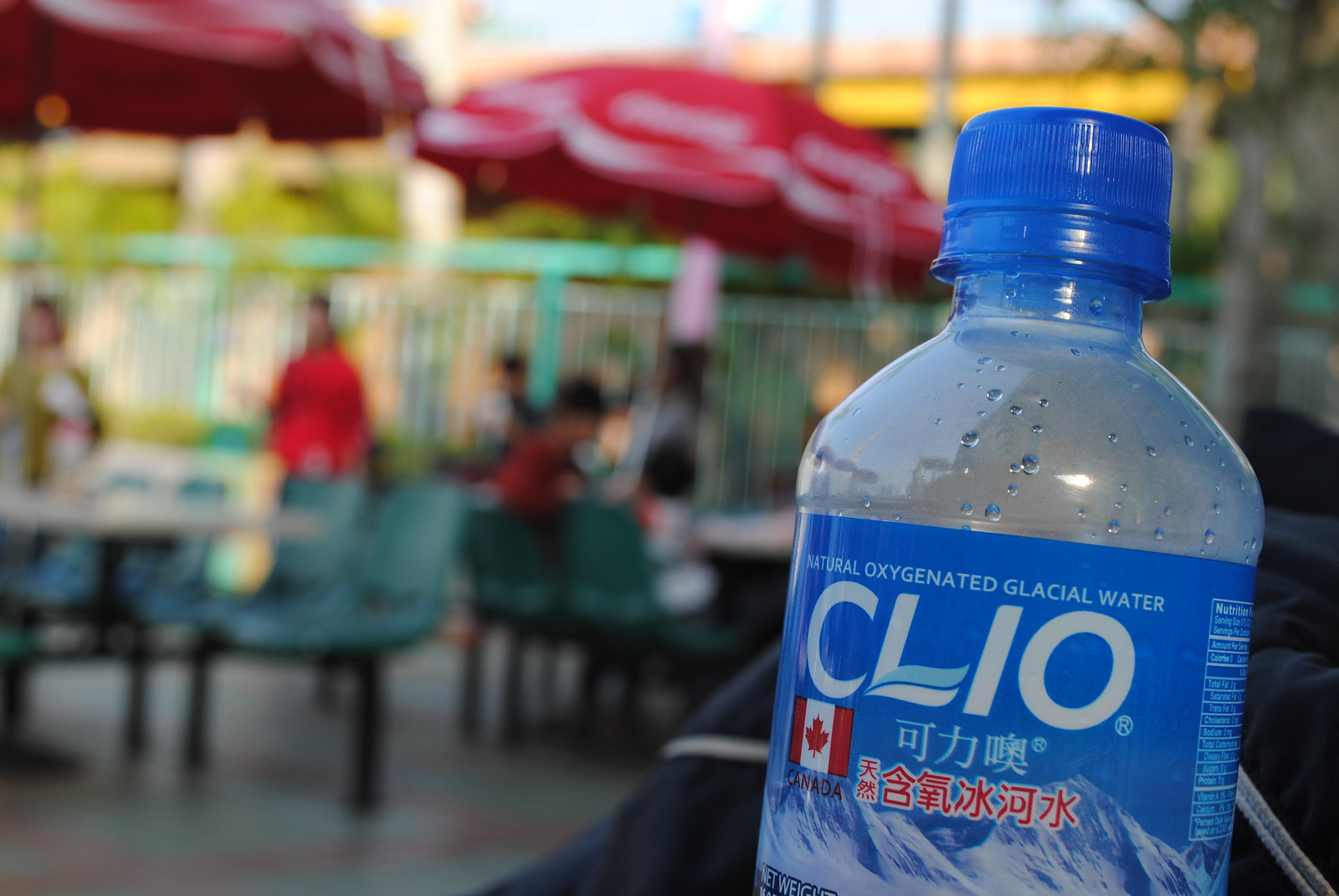The photograph features a close-up of the upper portion of a plastic water bottle. The bottle has a blue cap and a label with a blue background. Prominent English text on the label reads "Natural Oxygenated Glacial Water" and "CLIO." Below this, there's a Canadian flag and the word "Canada" in red. Accompanying this are two lines of Asian characters: three light blue characters on the first line and six red characters on the second line. To the right, near where the bottle curves, is nutritional information. The water in the bottle appears to have been drunk, as evidenced by visible condensation and water droplets near the top, below the cap.

The background of the image is very blurred, but it suggests an outdoor setting, possibly in a courtyard. There are tables and green chairs, and two red umbrellas with white writing are visible. A green fence with vertical bars can also be faintly seen, along with a yellow building in the distance. The scene appears to be within a social or recreational area, adding context to the setting of the photograph.